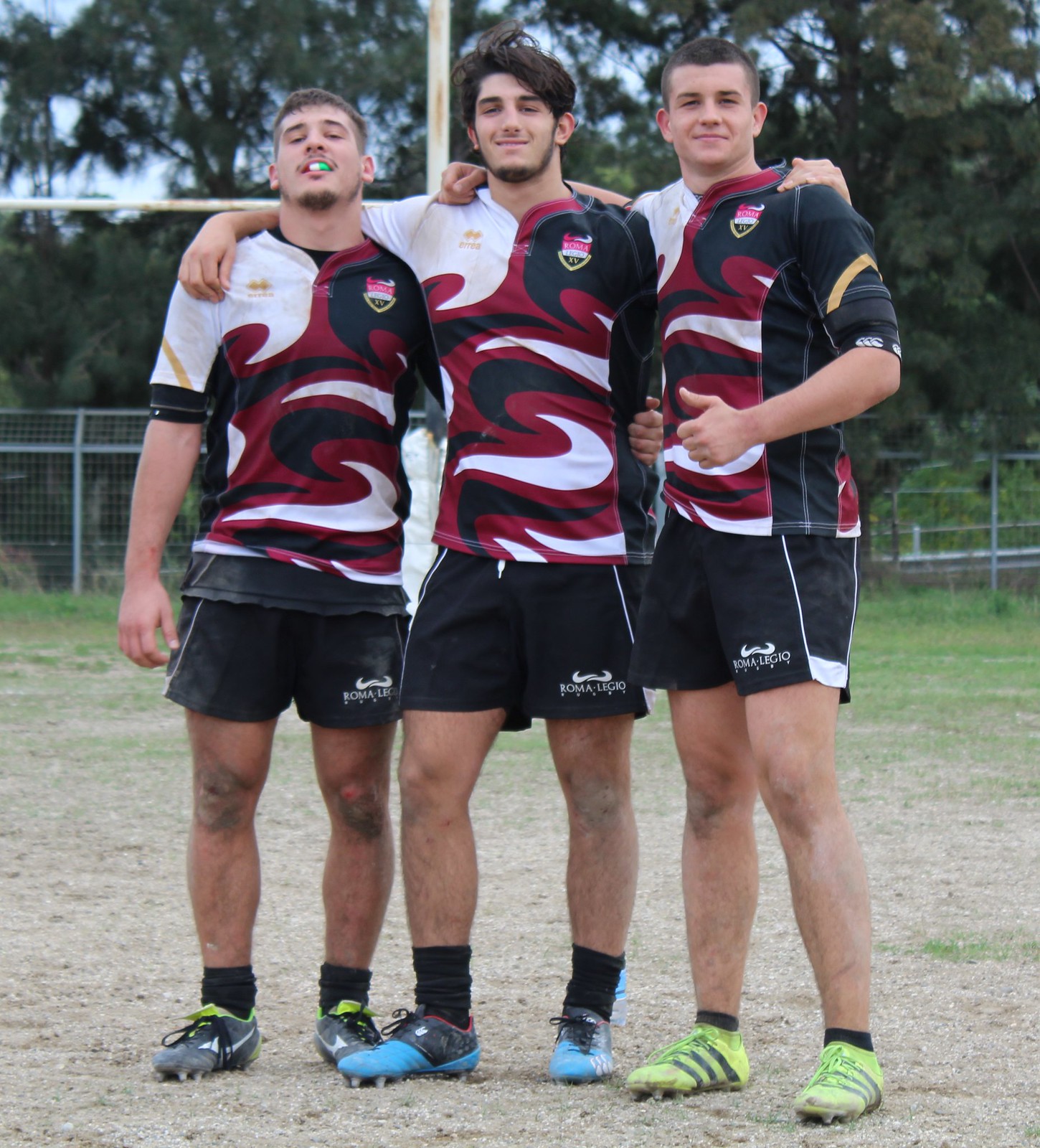In this photograph, three young boys, around 16 or 17 years old, stand side by side, arms around each other's shoulders, posing as if they have just won a game. They appear to be soccer players dressed in matching uniforms, featuring a distinctive swirl pattern in dark red, black, and white. Their shoulders are white and black, and their shorts are black with the inscription "Roma Legio" at the bottom. Each boy wears black ankle socks and cleats of various colors. The boy on the left sports an Italian mouth guard, while the boy on the right gives a thumbs up to the camera. They all have short hair and a muscular build, likely from their athletic activities. The setting is a mixed field of green grass and dirt, bordered by a silver chain link fence. In the background, tall green trees are visible against a clear blue sky, indicating it is daytime.